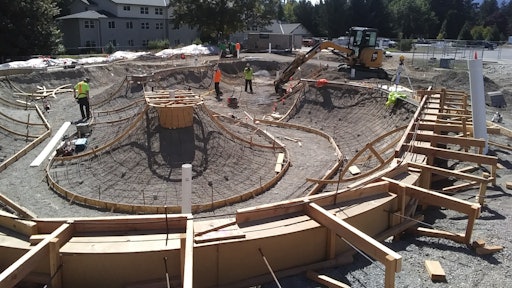In this photograph taken outdoors on a sunny day, a construction site is prominently featured in a horizontally rectangular frame. At the bottom left, a wooden wall stretches from left to right, gradually curving upwards and slightly rightward past the center. This wall features wooden supports extending outward and down to the ground.

At the focal point of the image, a large, circular indentation has been dug into the dirt. Within this excavation lies a central mound, fortified by wooden braces, with ropes or wires extending from the structure to its base. Surrounding this mound is a short, wooden frame border that encloses the middle area. 

Several workers in bright yellow and orange high-visibility shirts are seen standing around the site, engaged in construction activities. A digger or bulldozer, positioned towards the right, actively digs in the area, with its arm extended above the hole, contributing to the ongoing construction.

In the distant background, to the left, a large, gray multi-story house stands tall, flanked by lush green trees. Additional buildings and more verdant trees are visible further to the right, completing the scene. This detailed portrayal captures the industrious atmosphere of a sunny construction day, possibly for a future swimming pool, fountain, or a similar structure.